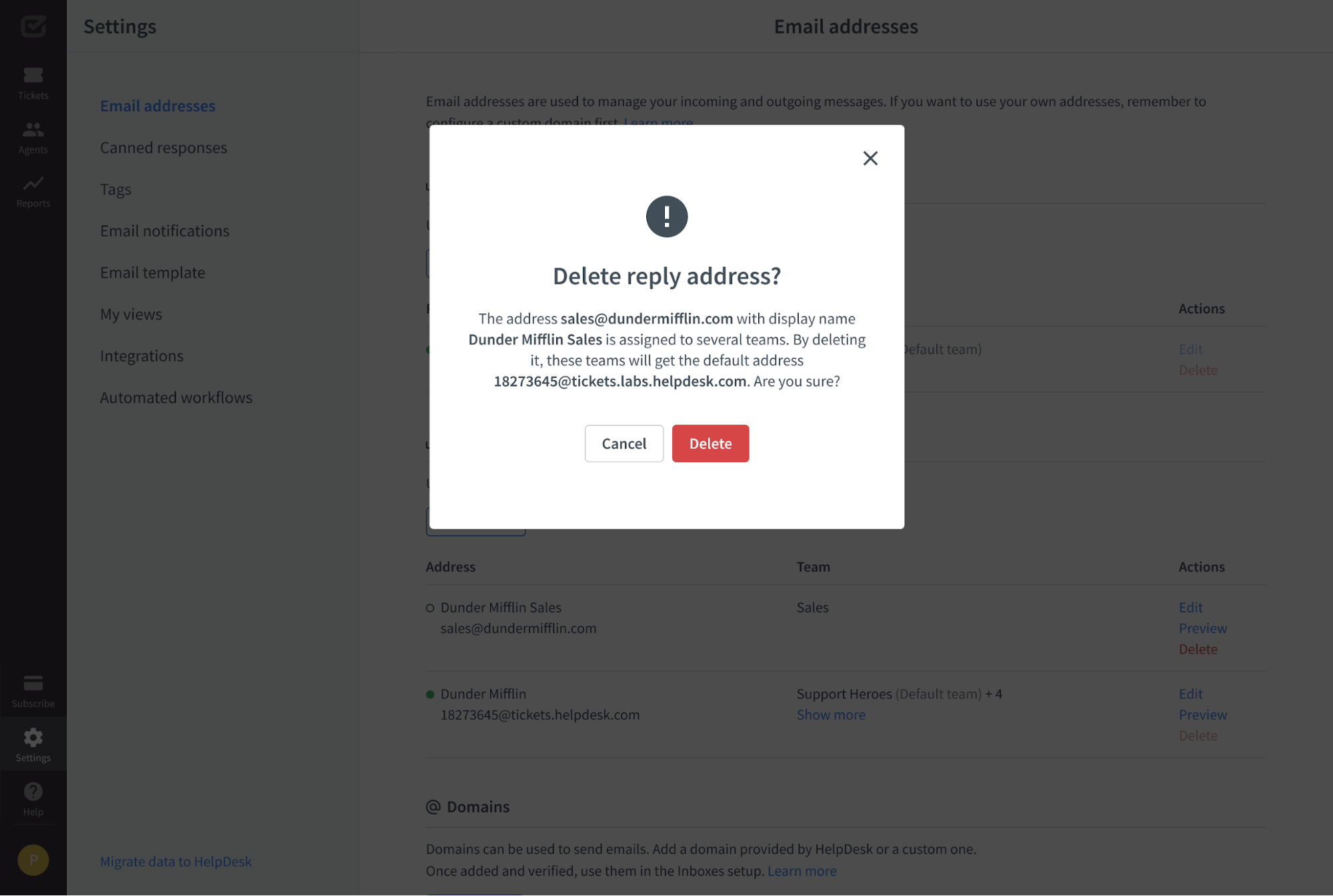Screenshot of Helpdesk Webpage

The screenshot portrays a section of a helpdesk webpage with a dark gray background. On the left-hand side, there's a slim vertical bar in a darker shade. The top navigation panel features options such as "Tickets" (accompanied by a ticket logo), "Agents" (illustrated with an icon of two people), and "Reports" (represented by a chart graphic). Towards the bottom of this panel, there are additional buttons including "Subscribe" (depicted with a credit card image), "Settings" (symbolized by a gear icon), and "Help" (marked by a circle with a question mark).

On the right-hand section under "Settings," various options are listed: "Email Addresses," "Canned Responses," "Tags," "Email Notifications," "Email Template," "My Views," "Integrations," and "Automated Workflows." At the top of this section, it reads: "Email Addresses," followed by an incomplete text: "Email addresses are used to manage your incoming and outgoing messages. If you want to use your own addresses, remember to..."

In the middle of the page, a prominent white box contains a deletion confirmation message: "Delete Reply Address." It mentions that the address "sales@dundermifflin.com" with the display name "dundermifflin sales" is currently assigned to several teams. Deleting this address will result in these teams being reassigned to the default address "18273645@tickets.labs.helpdesk.com." A prompt concludes with the question, "Are you sure?" Below this message are two buttons; "Cancel" on the left and "Delete" on the right.